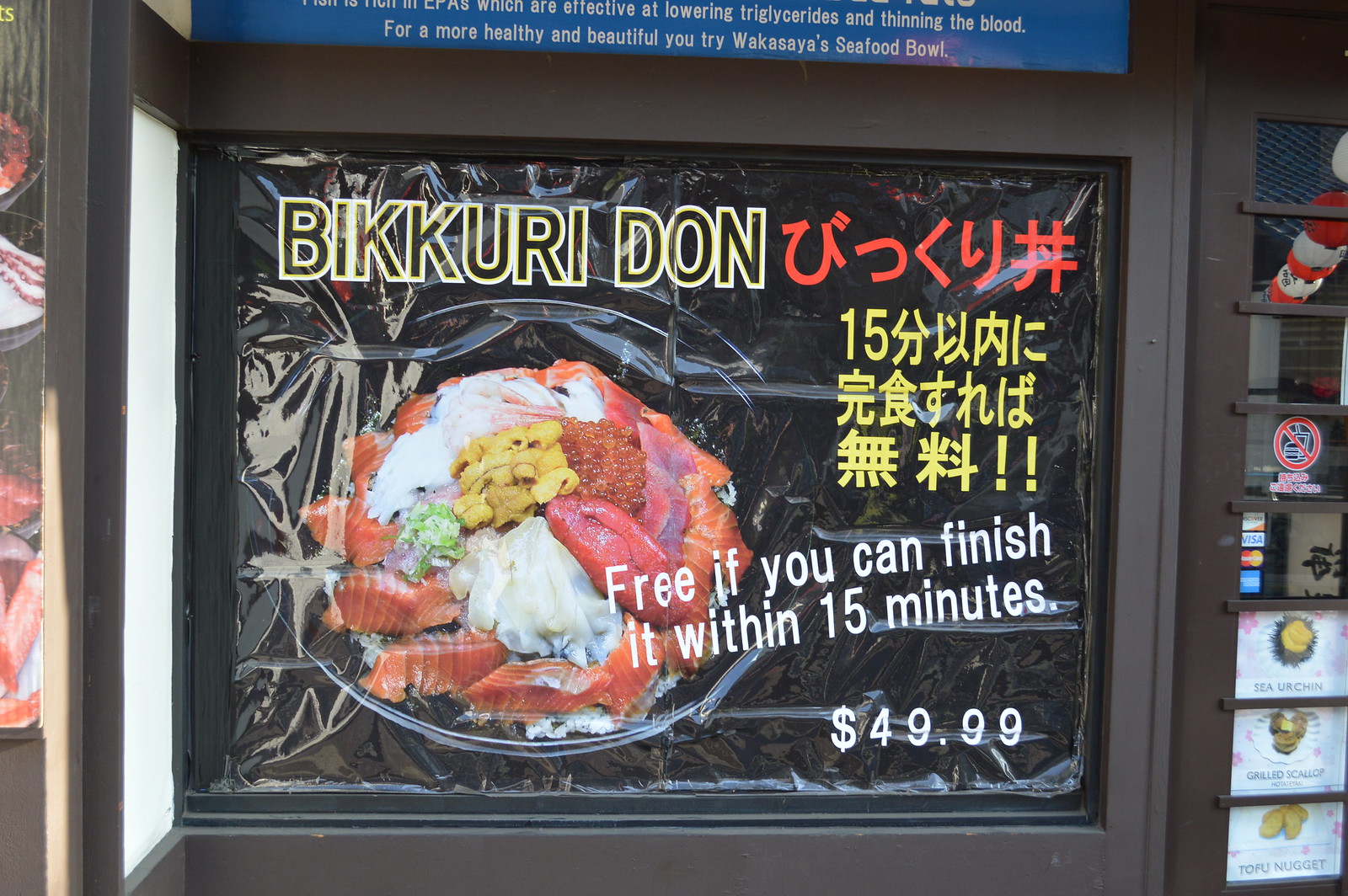This color outdoor daylight photograph captures an advertisement displayed in the window of a brown-painted storefront, likely a Japanese restaurant. The main feature is a large black sign that prominently showcases a substantial plate of seafood, including lobster and other varieties. Above the plate are the words "Bikkuri Don" in bold yellow letters, with accompanying non-English text, possibly Japanese, in red. A block of yellow text also in non-English appears above and around the number "15," hinting at the main challenge. Below the image of the food in white text, it clearly states, "Free if you can finish it within 15 minutes," alongside a price of $49.99. Surrounding the window are additional advertisements for menu items like sea urchin, grilled scallop, and tofu nugget. Nearby, there is a door with vertical slats and various stickers indicating credit cards accepted, including Discover, Visa, MasterCard, and American Express. The blue sign above the window features white text promoting health benefits, though it runs off the edge of the image. To the right of the door are signs forbidding smoking and outside food and drink.